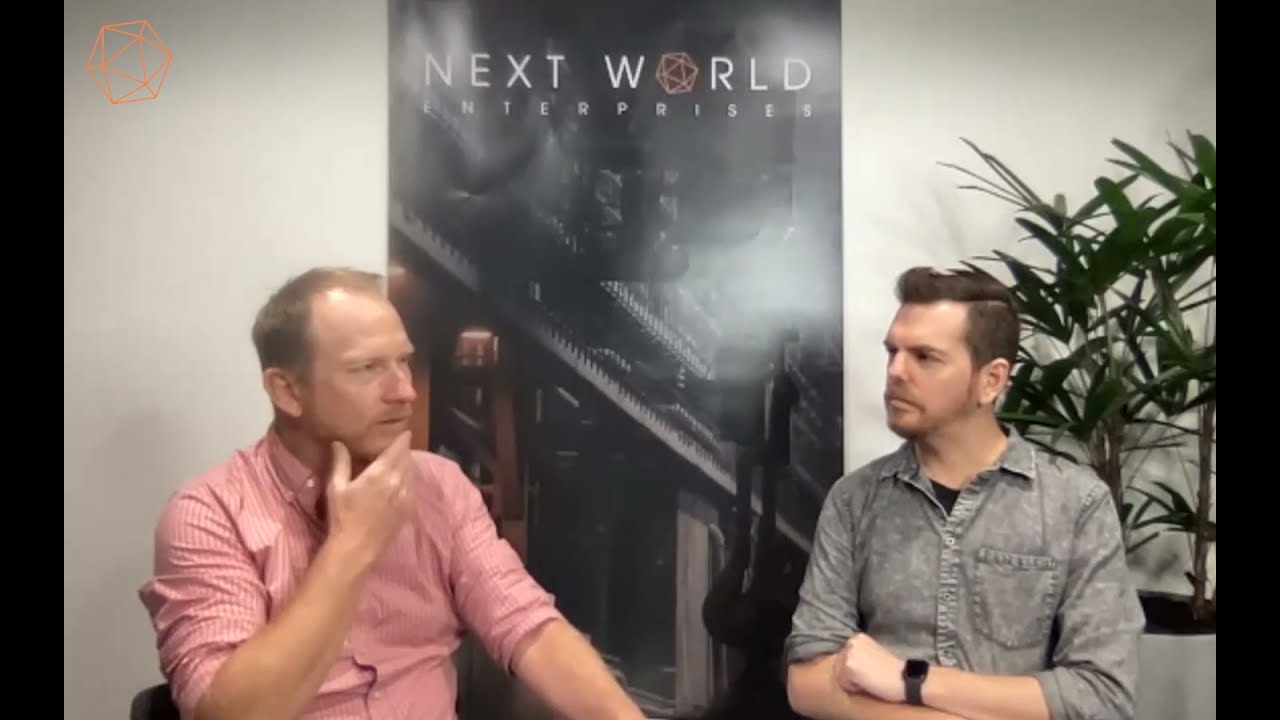In this image, a promotional interview or press release for Next World Enterprises is taking place. At the center, two white men are seated against a backdrop featuring a white wall and a prominent poster with the text "Next World Enterprises" in large white lettering. The letter "O" in "World" is creatively replaced by an orange geometric shape with triangles inside. On the top left of the backdrop, the same orange logo is visible. 

The man on the left appears to be in his mid-40s, with light brown, receding hair and a brown beard. He is wearing a red button-down shirt with the sleeves rolled up, and he has his hand on his chin in a thoughtful pose, seemingly giving an answer. His posture and expression suggest he is contemplating or explaining something.

The man on the right, likely in his late 30s, has short, darker brown hair with a light beard and mustache. He is dressed in a gray button-down shirt, also with rolled-up sleeves, and a black watch on his wrist. He seems to be the interviewer, looking towards the first man with his arms crossed, possibly waiting for a response. To his right is a vibrant green plant in a white pot, adding a touch of nature to the scene.

The image is framed by black borders on the very right and very left sides, enhancing the focus on the two men and the interview setting.